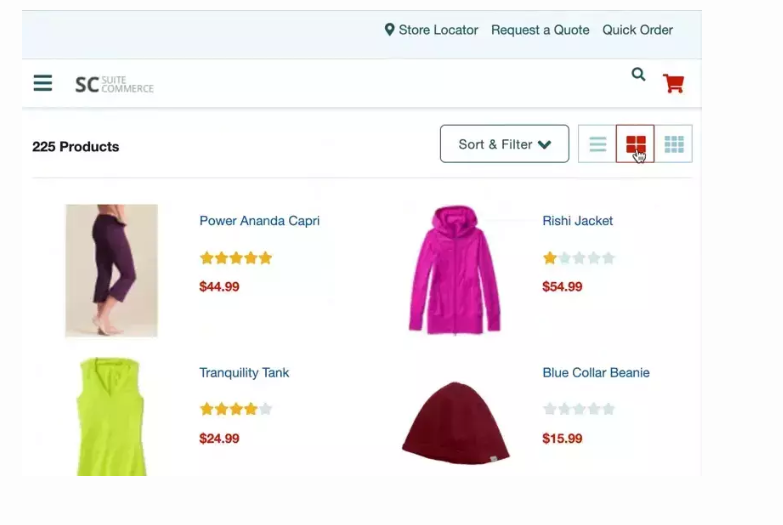The website I visited has a clean and organized layout with a light blue background. On the right-hand side, there's a teal map pin icon followed by the options "Store Locator," "Request a Quote," and "Quick Order." The background transitions to white, with a teal-colored section on the left featuring three horizontal lines. In dark gray text, it says "SC Street Commerce," and to the right, there's a teal magnifying glass icon, a red shopping cart, and a thin gray leaf. To the left, in black text, it notes "225 products."

A prominent white rectangle bordered in teal displays the options "Sort By," with a symbol for sorting accompanied by a downward arrow, and a filter icon represented by a teal box with three horizontal lines. Next to it, there’s a red-highlighted section with four squares, indicating the selected grid view. A white glove mouse cursor is clicking on this red-highlighted grid.

Below, the products are showcased:

1. On the left, in teal, it says "Power Ananda Capri" rated with five red stars, priced at $44.99. A person is shown wearing burgundy Capris.

2. Next, "Tranquility Tank" with four stars in red, priced at $24.99, displayed on a green tank top.

3. Then, a "Rishi Jacket" with a teal label rated one star in red, priced at $54.99, shown in pink.

4. Lastly, an item named "Blue Collar Beanie," although the beanie itself is red with no stars displayed, has its description in teal and the price in red at $15.99. The text and stars for this item are in gray.

This layout provides a vibrant, user-friendly interface for browsing the available products.